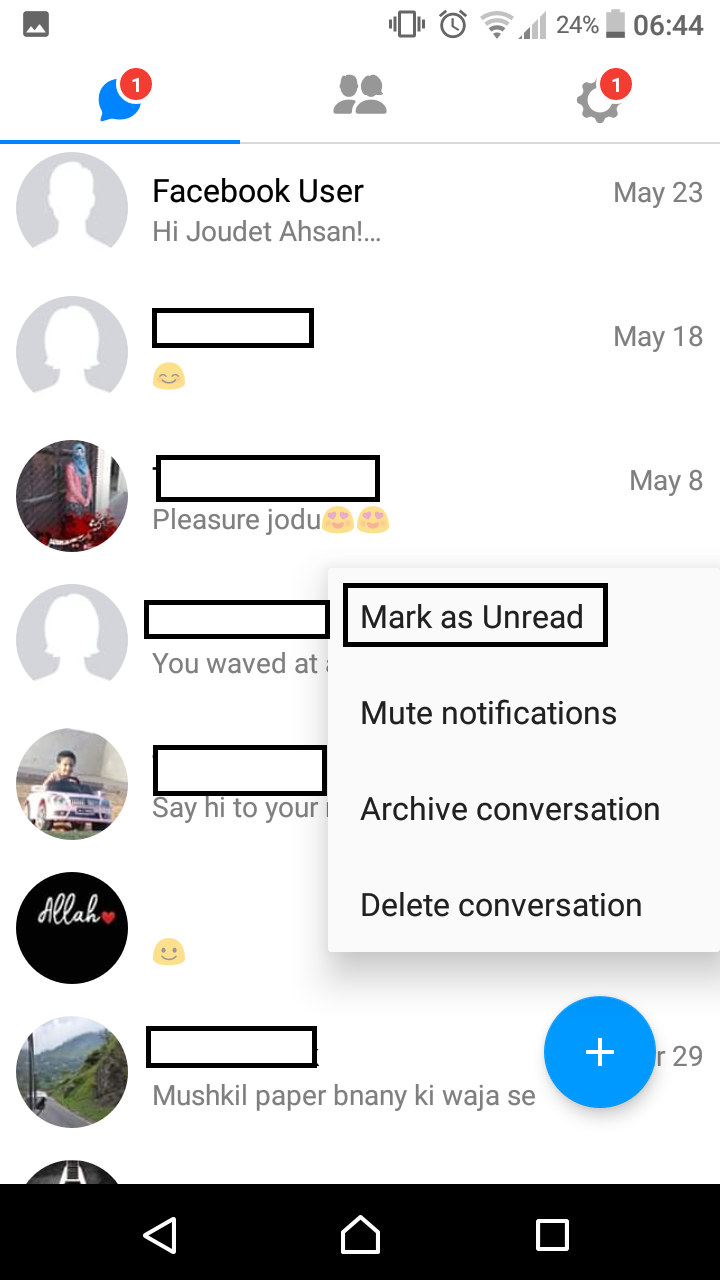The image is a screenshot of multiple messages within the Facebook app. The first message displays the username as "Facebook User," and the content reads "Hi Jodette Ahsan." This message is dated May 23rd. Subsequent usernames have been obscured, and the next message, dated May 18th, consists solely of a smiley face emoji. The following message, dated May 8th, says "please shoru" accompanied by two heart-eyes emojis. Additionally, there is a pop-up window on the right side of the image. The first option in this window, highlighted with a black stroke, reads "Mark as Unread."